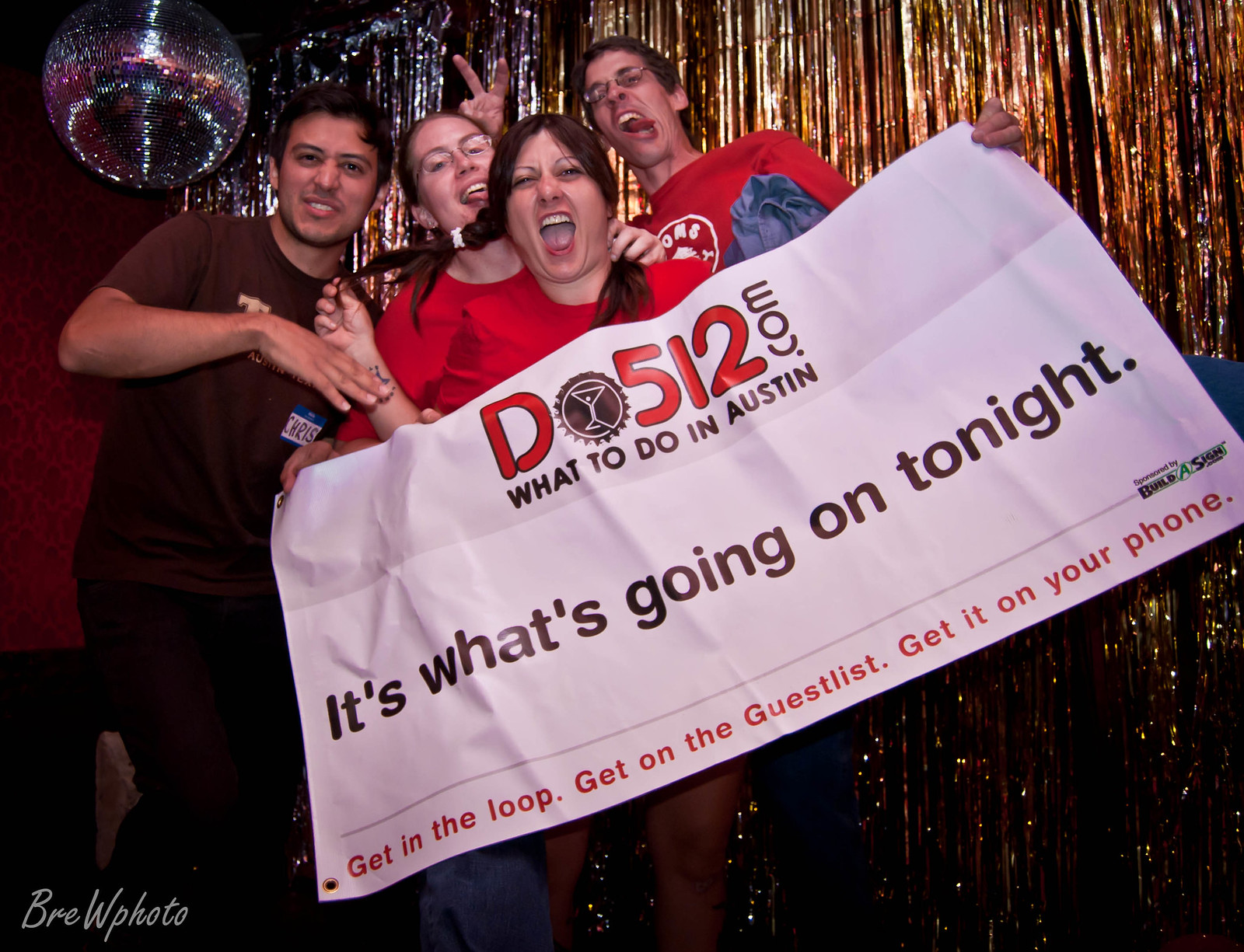This vibrant photograph captures four lively individuals promoting the website do512.com. The central figure is a woman with long brown hair, wearing a red shirt and pigtails, holding a banner that reads "do512.com. What to do in Austin. It's what's going on tonight. Get in the loop. Get on the guest list. Get it on your phone," with a sponsorship note stating "Sponsored by Build A Sign." Behind her, a silver and gold tinsel curtain, with a disco ball in the upper left and a credit to Brie W Photo in the lower left, creates a festive atmosphere.

To her left stands a young man in a brown shirt with tan skin and black hair, sporting a neutral expression. To her immediate right, another woman in a red shirt sticks out her tongue and wears glasses, making a funny face. The far-right figure, a second man also in a red shirt, is donning glasses and making a humorous expression while gesturing with bunny ears behind the woman with glasses. All four appear joyous and energized, seemingly celebrating and cheering together. Their open mouths and animated gestures suggest they are thrilled to promote the event listed on the banner.